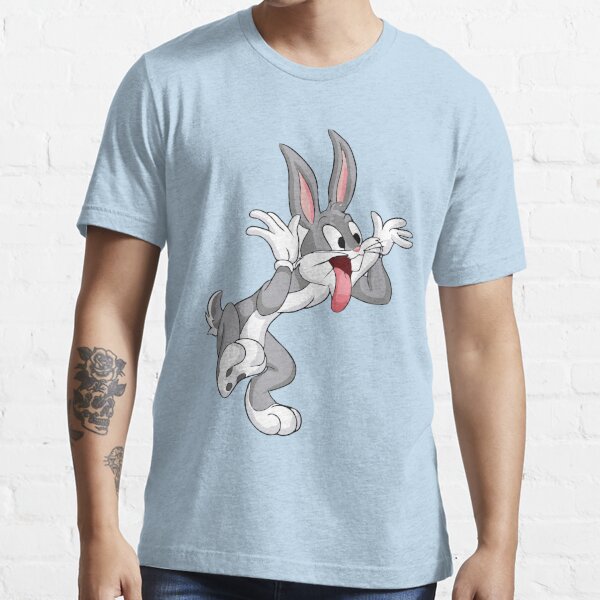In this image, we see a male model standing against a white brick wall, wearing a light blue, heather-colored t-shirt. The t-shirt prominently features a playful cartoon depiction of Bugs Bunny. The iconic character is depicted standing on his left foot, with his right leg lifted in the air, and his tongue sticking out towards the right side of his mouth in a teasing manner. His hands are positioned by the sides of his head, as though waving or playfully challenging someone to catch him. Bugs Bunny’s gray ears stand straight up with the pink interior visible, complementing the pink of his tongue.

The photograph is framed in such a way that the man's head is cropped out, focusing attention on the t-shirt and his upper body. His arms, which hang naturally by his sides, are both exposed. Notably, the model's right forearm features detailed tattoos: a blue flower design on the forearm, a skull with a flower coming out of it just below the shoulder, and additional tattoo elements extending closer to the wrist. The bottom of the image captures the top of his blue jeans, adding to the casual style presented in the photo.